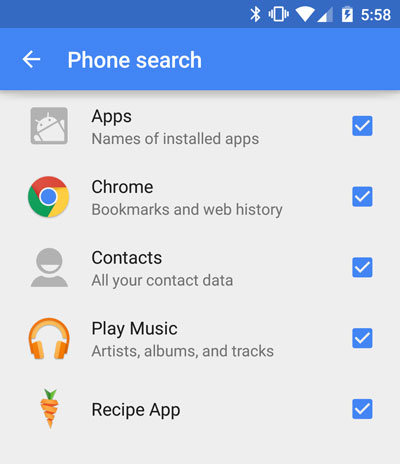**Descriptive Caption:**

This image is a partial screenshot captured from a cell phone screen. At the top of the screenshot, you can see a dark blue status bar. The status bar displays several icons on the upper-right corner: a Bluetooth icon, a phone icon, a Wi-Fi signal icon indicating two out of four bars, and a battery icon. The battery is fully charged and features a blue lightning bolt in the center. The time displayed is "5:58." Directly below the status bar, a lighter shade of blue background holds a white back arrow and the text "Phone Search."

The main section of the screenshot features a gray background with a column of app icons on the left side, each accompanied by a description on the right. Each line also includes a blue square checkbox with a white checkmark inside on the far right. 

The app icons and their descriptions are as follows:
1. A small gray Android square with a white Android icon – labeled "Apps, names of installed apps."
2. The Google Chrome icon – labeled "Chrome, bookmarks and web history."
3. A human silhouette icon in gray – labeled "Contacts, all your contacts data."
4. A set of orange and yellow headphones – labeled "Play Music, artist albums and tracks."
5. An orange and green carrot icon – labeled "Recipe Apps."

This image seems to be taken from a settings or management application likely used for organizing or backing up app data on the phone.